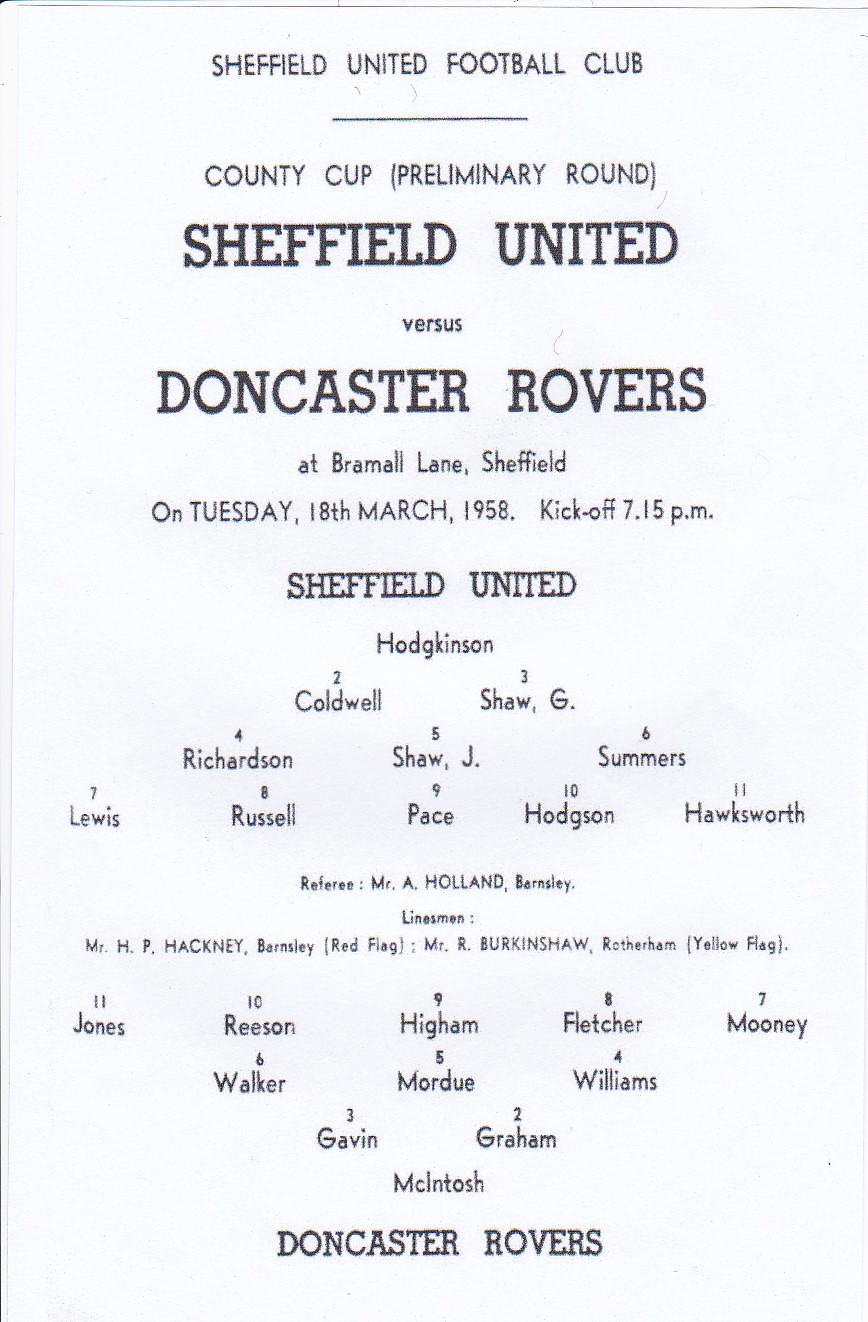This image is a vintage program from a historic football match. At the top, it prominently reads "Sheffield United Football Club County Cup Preliminary Round, Sheffield United versus Doncaster Rovers at Bramall Lane, Sheffield, on Tuesday, 18th March 1958, kickoff at 7.15 p.m." The text provides details of both teams' lineups for the match. 

For Sheffield United, the players listed are: Hodgkinson (goalkeeper), Caldwell, G. Shaw (defenders), Richardson, J. Shaw, Somers (midfielders), and Lewis, Russell, Pace, Hodgkinson, Hawksworth (forwards). The match officials included Referee Mr. A. Holland from Barnsley, with Linesmen Mr. H.P. Hackney from Barnsley holding the red flag, and Mr. R. Birkinshaw from Rotherham holding the yellow flag.

The opposing team, Doncaster Rovers, featured McIntosh (goalkeeper), Gavin, Graham (defenders), Walker, Mordew, Williams (midfielders), and Jones, Rison, Higham, Fletcher, Mooney (forwards). This setup likely suggests the hierarchical arrangement of teams and matches leading to this event, possibly depicted at the bottom in a tournament bracket style.

Overall, the document encapsulates a detailed snapshot of a significant match, providing a full roster and official details that contribute to its historical narrative.